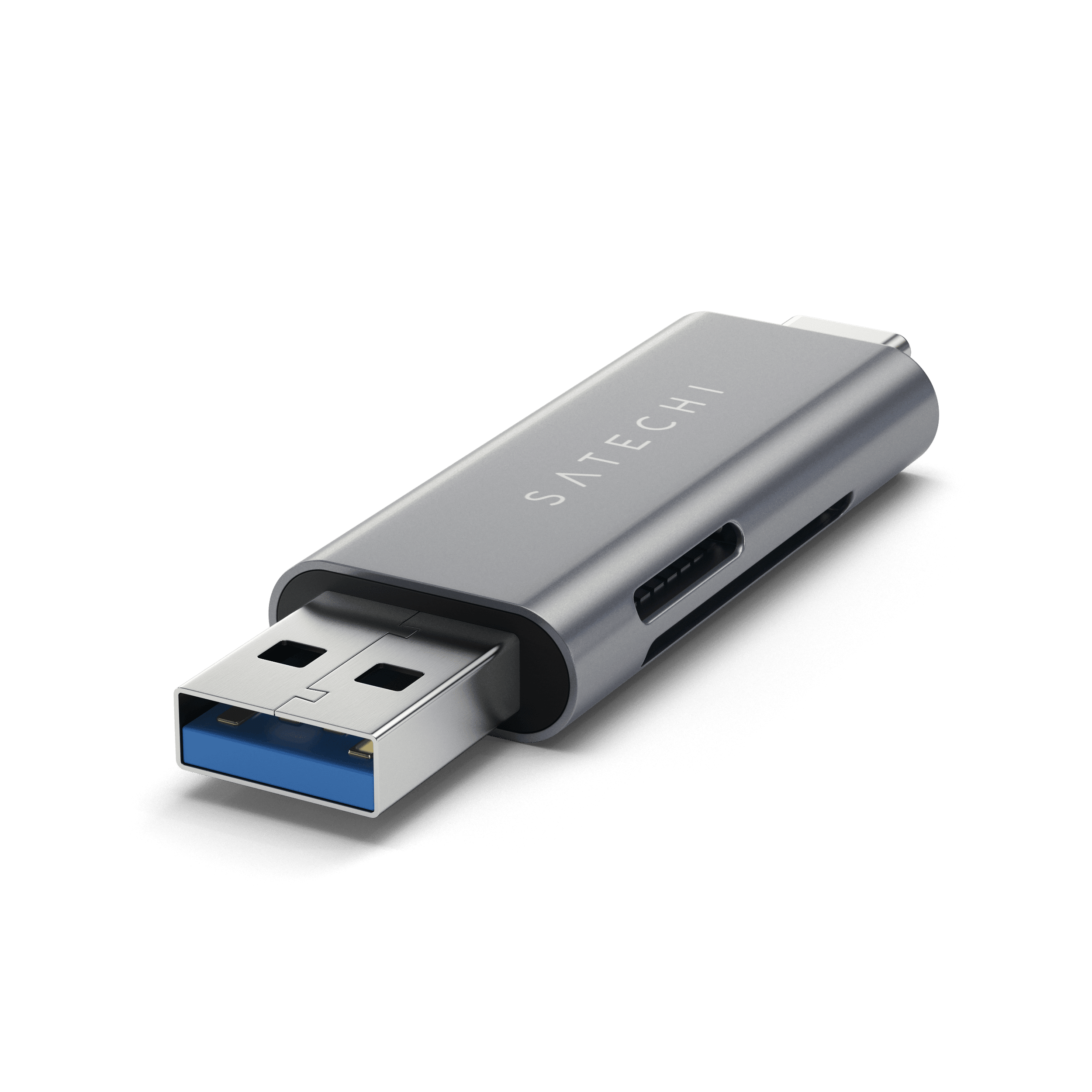The image features a single USB drive positioned on a white background. The drive is silver in color with its top cap removed, revealing the blue metallic part that inserts into the computer. Oriented with the top facing down towards the bottom left and the bottom facing up to the top right, the USB drive has "Satechi" embossed on its surface, spelled out as S-A-T-E-C-H-I. The exposed USB connector has two small square holes carved into it. The drive appears designed to potentially allow another USB connection on the opposite end, evident from its multiple openings and the metallic extension on the back.